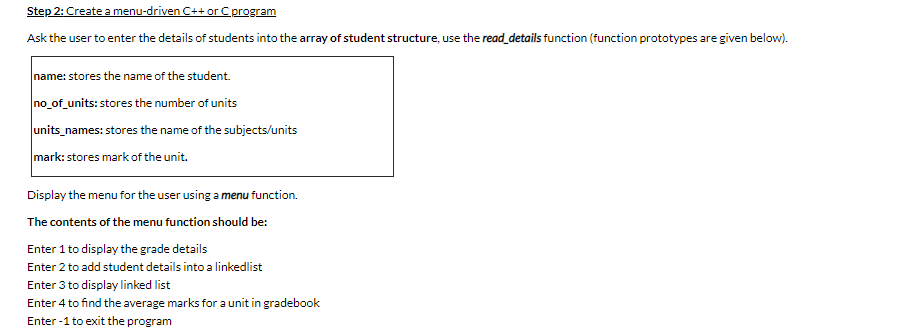A set of instructions is presented on a white background. At the top, "Step Two" is prominently bolded and underlined in black. Following that, the instructions read: "Create a menu-driven C++ or C program."

The document specifies that the program should prompt the user to enter the details of students into an array of student structures. A function named `road_details` is highlighted in bold, indicating its use in the program.

Additionally, there are function prototypes mentioned below in a bracketed print. Inside a delineated box, details of various elements of the student structure are listed:
- `name`: stores the name of the student
- `number_in_all_of_the_units`: stores the number of units
- `units_names`: stores the names of the students/units
- `mark`: stores the mark of the unit

The instructions proceed to emphasize displaying a menu for the user through a menu function. The menu function's contents are described sequentially:
1. Enter 1 to display the grade details.
2. Enter 2 to add the student details into a linked list.
3. Enter 3 to display a linked list.
4. Enter 4 to find the average marks per unit and grade book.
5. Enter -1 to exit the program.

The instructions conclude without any additional information beyond the aforementioned guidelines.